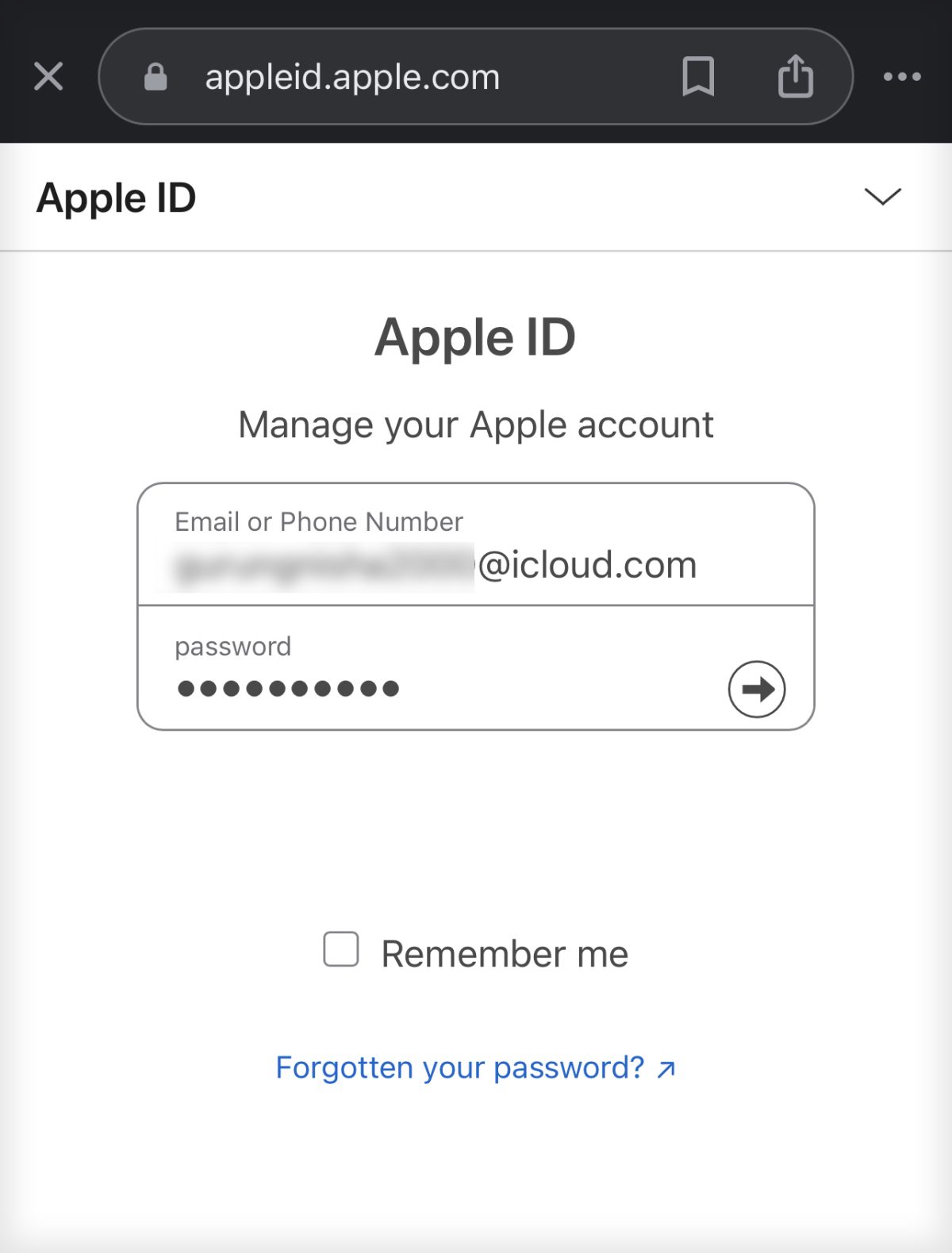The image depicts a web browser interface, specifically an Apple ID login page. At the top, there is a black bar with an X on the left, followed by a search bar that contains a padlock icon and the URL "appleid.apple.com." Next to the search bar are bookmark options, a box with an upward arrow, and three horizontal dots.

Below this bar, the main content of the page appears against a white background. On the left, it starts with "appleid" featuring a dropdown menu represented by a small arrow. Adjacent to this, in a centered position, is the title "appleid," followed by the subtitle "Manage your Apple account."

The login form is prominently displayed, beginning with fields for either an email or phone number. The entered text in this field has been blurred for privacy, and the domain "icloud.com" is visible. Beneath this, the password field displays obscured characters. At the bottom-right corner of the password field, there is a circular arrow indicating the submission button.

A checkbox labeled "Remember me" appears under the login fields, which is currently unchecked. Further down, a blue text link reads "Forgotten your password?" with a diagonal arrow pointing to it.

The color scheme of the page primarily includes black, white, gray, and blue, maintaining a clean and simple aesthetic to enhance readability and focus.